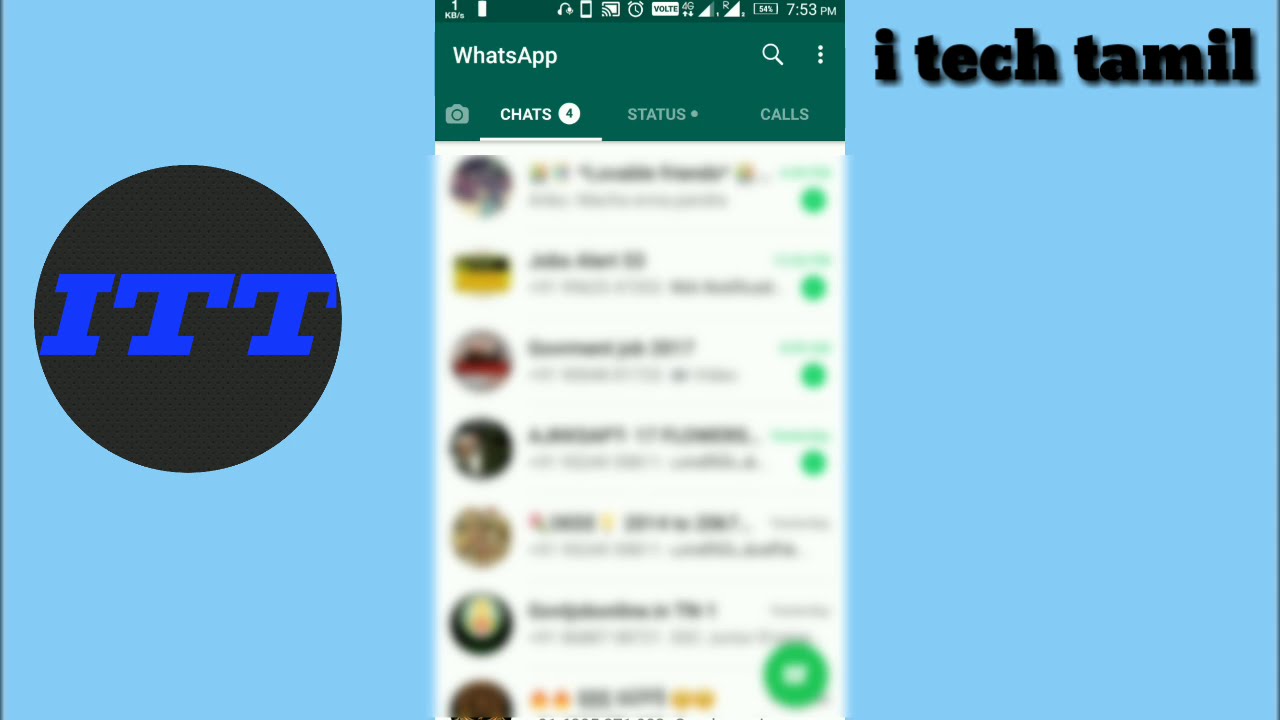The image depicts a computer screen with a light blue background. A gray circle with the blue capital letters "ITT" is prominently positioned on the left side of the screen. Meanwhile, the top right corner features the text "iTech Tamil" in lowercase black letters. Centrally, the screen resembles an open WhatsApp application, displaying the interface of a phone screen, albeit without the actual phone being visible. At the top of this phone-like interface, "WhatsApp" is written in white, along with the time "7.53 p.m." To the right of the clock are three dots and a magnifying glass icon. Below are tabs for "Chats," which lists "4" unread messages, "Status" with a green dot, and "Calls." Below these options, at the bottom of the page, there's a camera icon, accompanied by an area that appears blurred and unreadable. The overall presentation is clean yet detailed, capturing the primary elements without the distractions of the blurred section at the bottom.